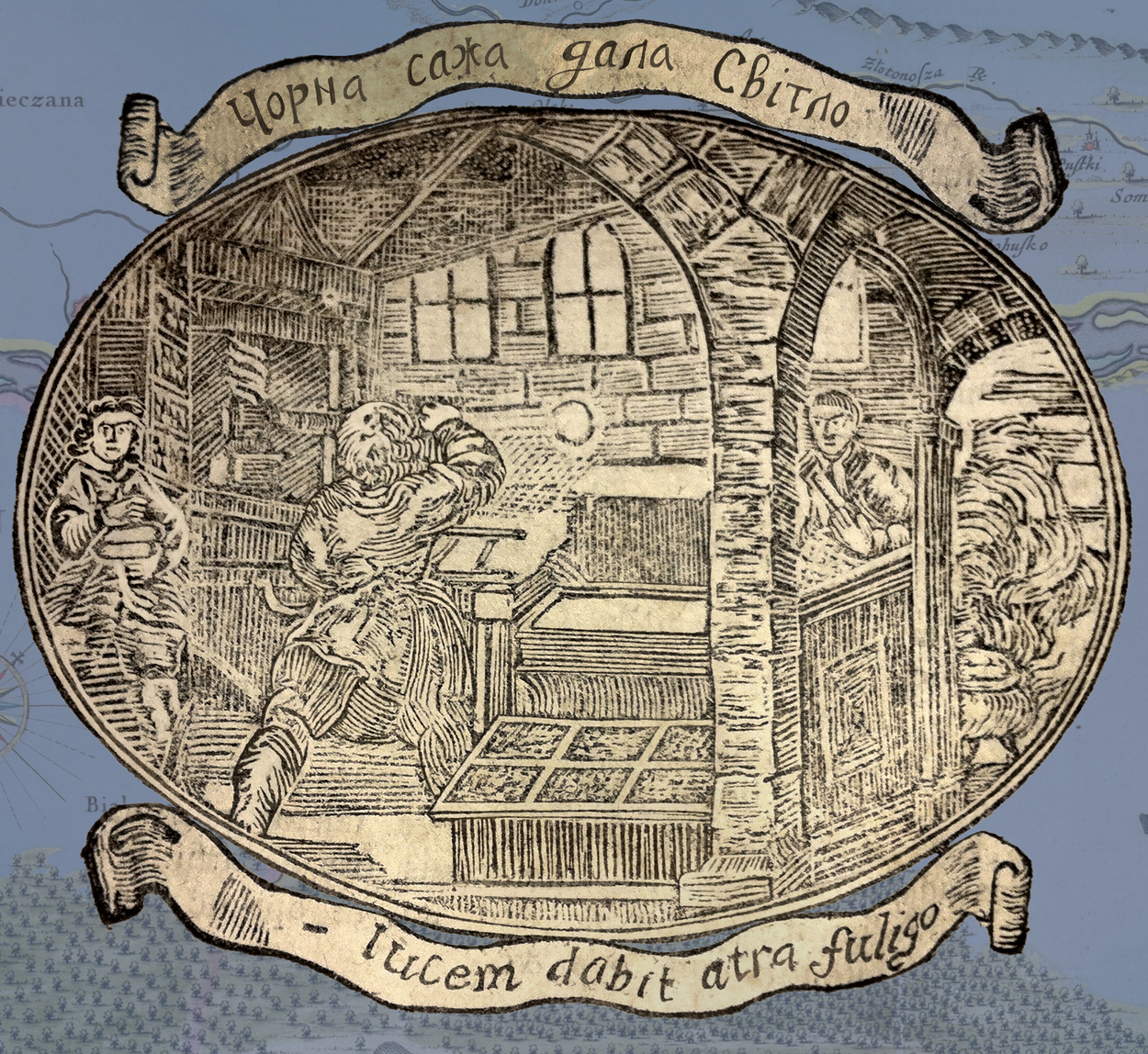The detailed black-and-white illustration, reminiscent of an old sketch from perhaps the post-medieval period, depicts a scene set within a workshop or similar indoor setting. The artwork emphasizes intricate hand-drawn lines, capturing the essence of a bygone era, likely the 14th or 15th century. Three men, dressed in period clothing with distinctive old-style haircuts, interact amidst shelves and boxes, suggesting a busy environment. Surrounding the scene are two banners – the top one featuring indecipherable text in a foreign language, while the bottom banner is inscribed in Latin. The entire image sits against a tan or gray background with hints of blue, further enriched by faint black markings reminiscent of a map, imparting a historical and somewhat enigmatic aura to the illustration.